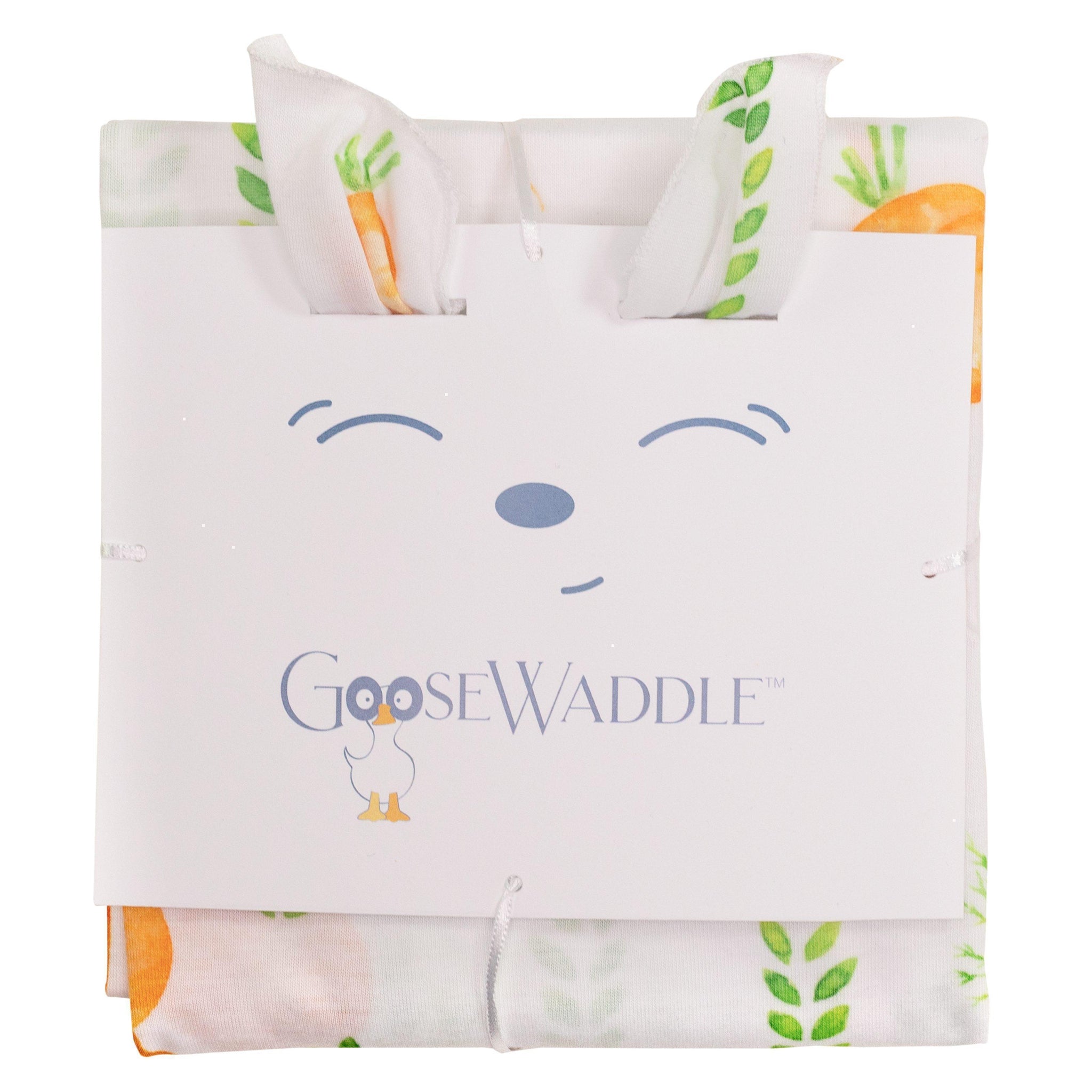This image features a baby swaddling set designed to look like a bunny. The packaging includes a white card that reads "Goose Waddle" in light blue text. Intriguingly, a cartoonish goose with a white body, yellow beak, and yellow feet peeks through the two O's in "Goose," using them as its eyes. Above the brand name is a whimsical drawing of a bunny-like face, featuring closed, slanted blue eyes, a small button nose, and a simple smiling line. 

The fabric of the swaddling set is white and adorned with a playful pattern of orange carrots with green leaves, adding a charming touch. The fabric has a slightly meshy texture, giving it a semi-transparent appearance. Part of the fabric is arranged to protrude through the card, resembling bunny ears, thus completing the adorable bunny-themed design.